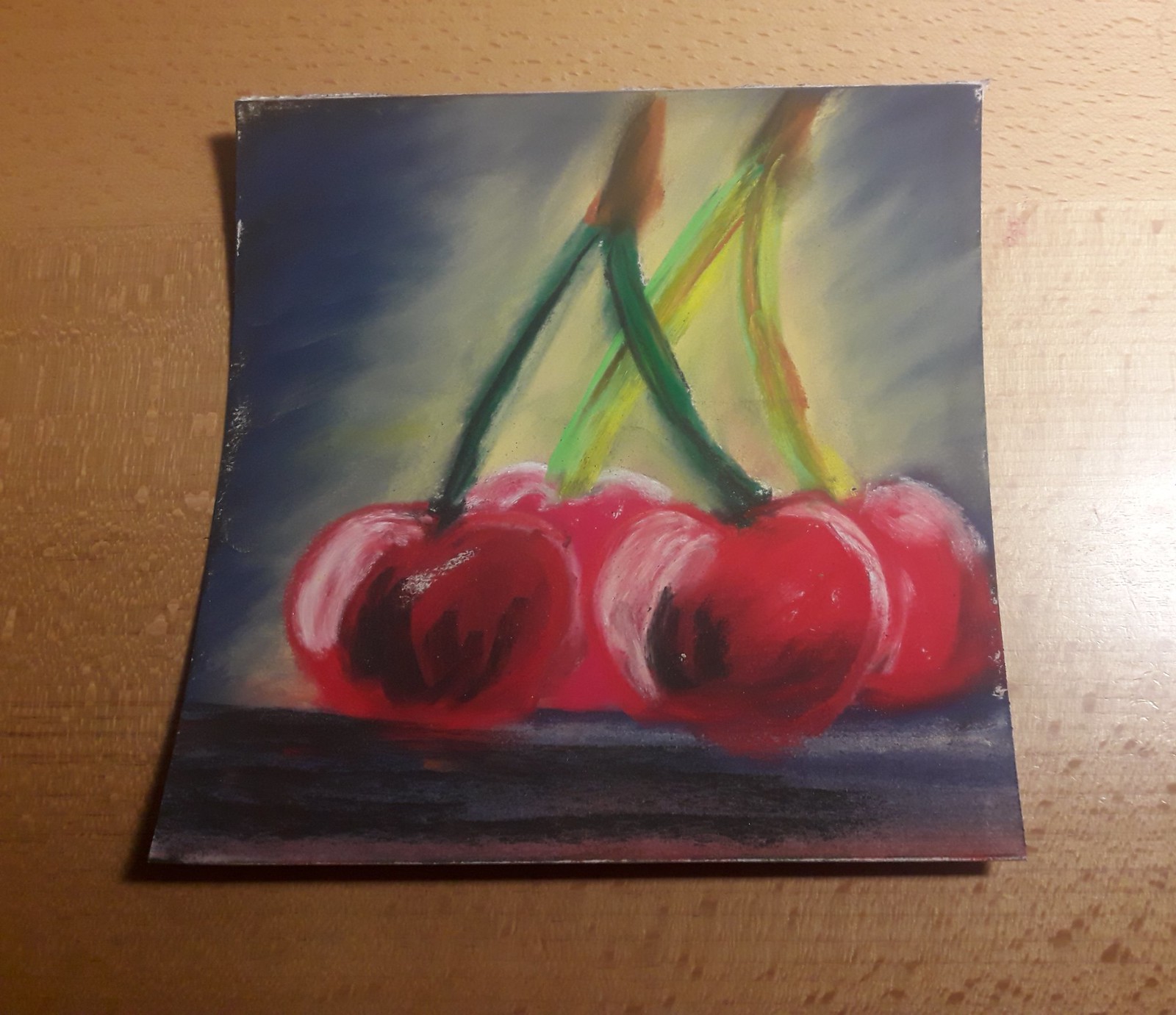This is a color photograph showcasing a close-up of an impressionistic painting displayed on a golden brown wooden surface, which brightens towards the right due to directed lighting. The painting medium, possibly slightly curved fabric or paper, features a depiction of cherries. There are three to four cherries, each rendered with rich red hues, enhanced with black shading and highlights. Light green stalks, some darker and intersecting at a central brown point in the foreground, and lighter yellowish-green stalks that converge in the background, suggest varying stages of ripeness. The cherries rest on a blue background, contrasted by a darker blue base. At the very bottom, a subtle red reflection hints at the cherries' glossy surfaces, adding a touch of realism to the impressionistic artwork.